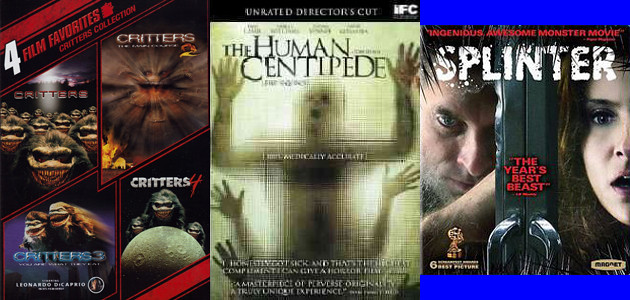The image features three distinct DVD covers, each showcasing a different movie or movie collection. On the far left is the "4 Film Favorites: Critters Collection," prominently displayed in red with a white "4." This cover includes the titles "Critters," "Critters 2," "Critters 3," and "Critters 4," all separated by red lines. In the center is the cover for "The Human Centipede," characterized by an eerie depiction of a person's silhouette pressed against what looks like an opaque window, with three pairs of hands visible on the surface. The title is written in black, and the top of the cover notes it as the "Unrated Director's Cut." On the far right is the cover of the movie "Splinter," which features a man on the left and a woman on the right. The title is prominently displayed in white, with blue bars at the top and bottom of the cover. Below the title, a red quote praises it as "The Year's Best Beast," and the lower right corner of the cover indicates that it is a Magnet release.